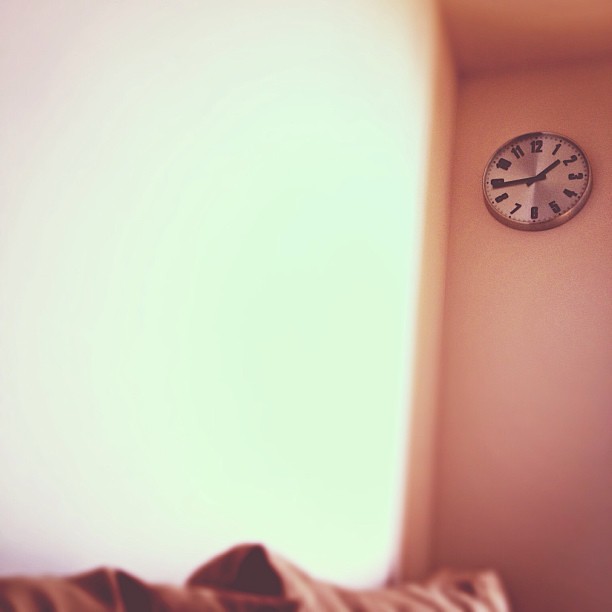In the image, a round clock with a silver border hangs on a smooth, light pinkish-beige wall, positioned towards the far right side of the frame. The clock features large black numbers from 1 to 12 and matching black hands, indicating the time as 1:44. Dominating the left side of the image is a corner, with an adjoining wall that is brightly illuminated, possibly by sunlight, giving it an almost white to light yellow hue. At the bottom of the image, the top of a plush couch or a stack of pillows is partially visible.